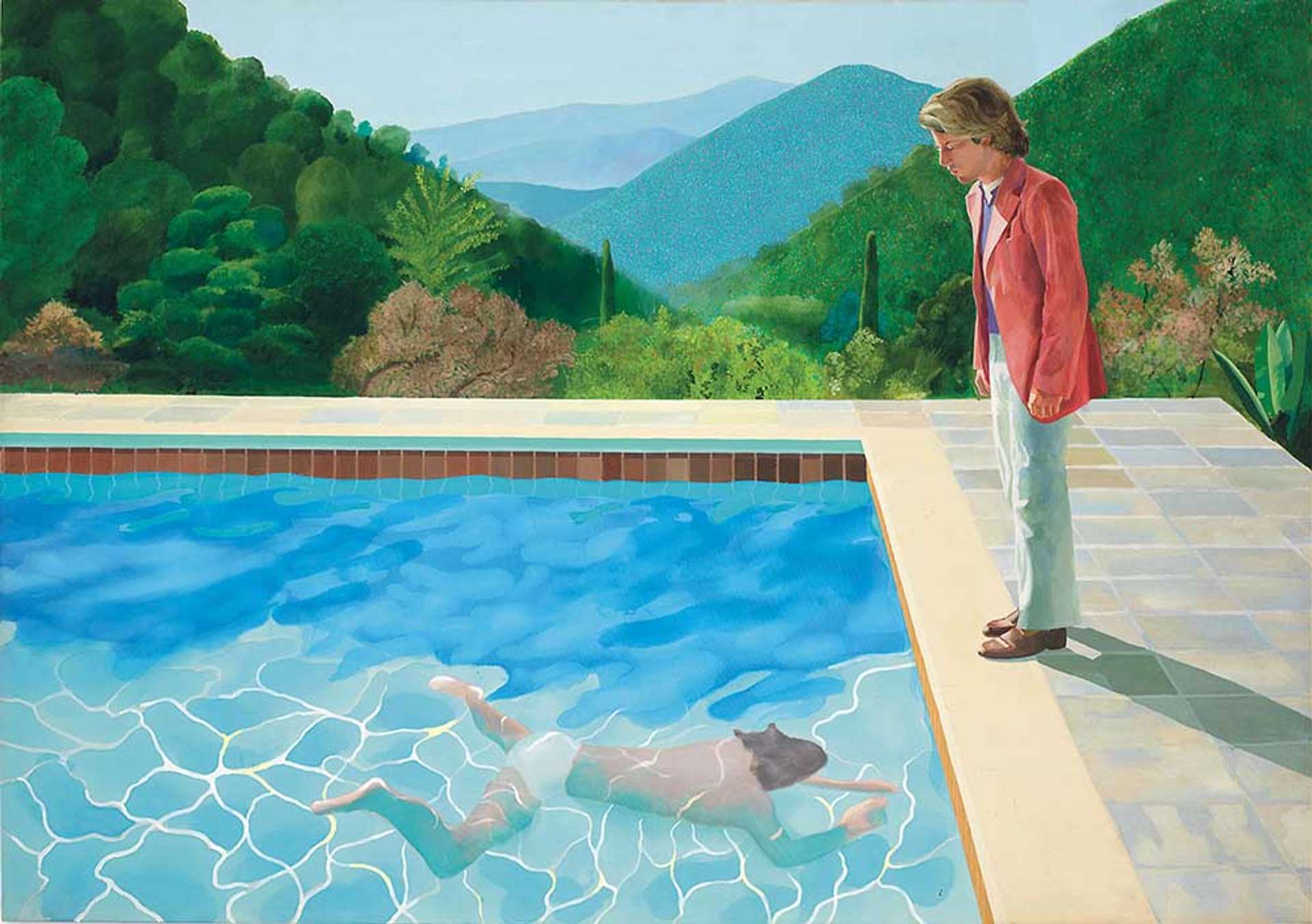This detailed watercolor painting depicts a serene yet enigmatic scene set in what appears to be the Hollywood Hills. The focal point is an in-ground pool surrounded by light tan and pastel purple tiles on the outer rim and red brick tiles lining the inner rim. The crystal-clear pool water mirrors the gentle hues of the surroundings.

On the poolside stands a young man, possibly in his twenties, who exudes an air of classic Hollywood style. He is dressed in a striking red-pink long-sleeved jacket over a purple shirt, complemented by white pants and brown leather shoes. His short, wavy brown hair frames his face as he gazes intently into the water. His expression is one of concern or contemplation, as he looks at the figure swimming below.

Underneath the water, a man with long dark hair swims leisurely. Clad only in white underwear, his form is gracefully captured mid-stroke, adding a touch of ambiguity to the scene—one might ponder if he is serenely swimming or perhaps in some distress, given the grave look from the man above.

In the distance, the painting captures the lush, rolling hills and distant mountains, evoking the tranquil and luxurious vibe of a secluded hillside retreat. The detailed elements and the emotionally charged interaction between the two figures suggest a narrative depth that makes the viewer wonder about the underlying story, possibly hinting at a scene from a movie adapted into this evocative painting.